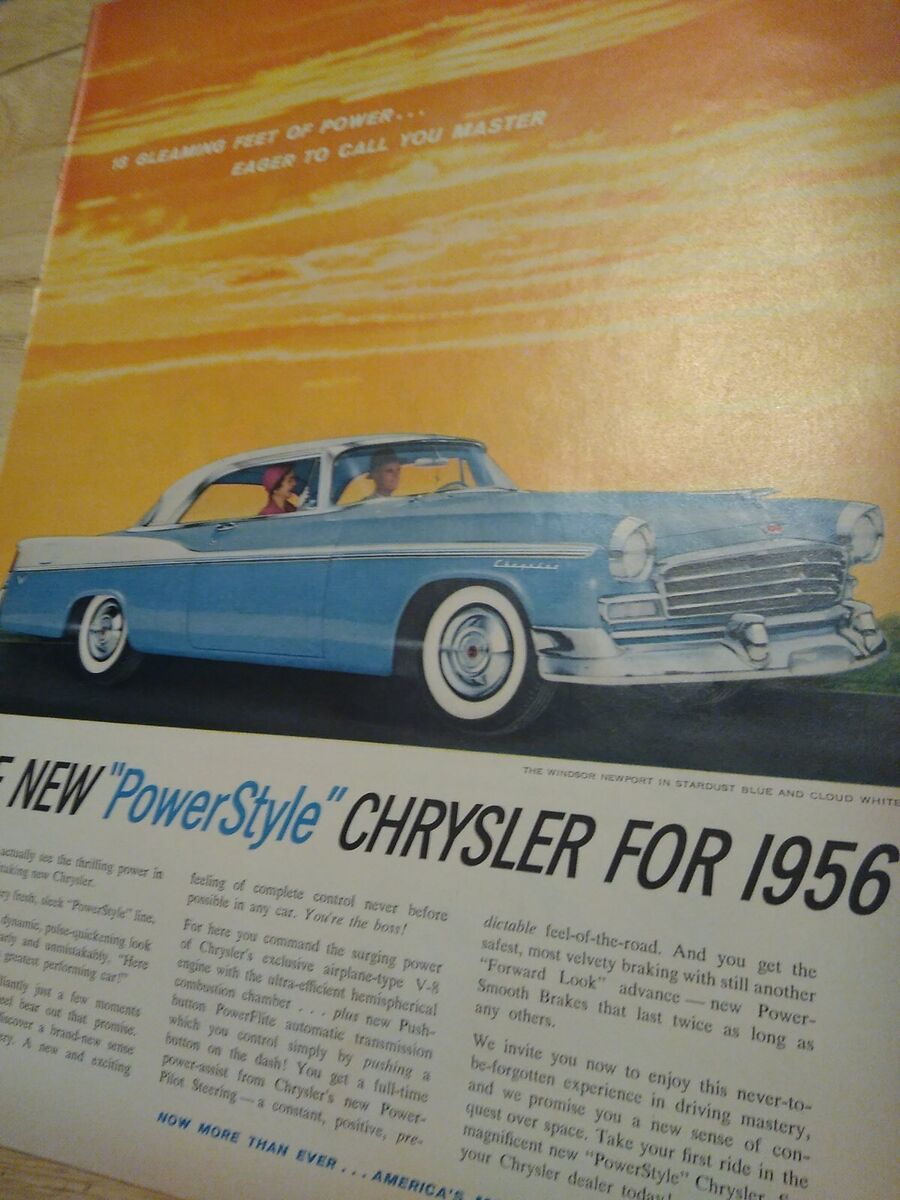The image is a vibrant vintage magazine advertisement for the 1956 Chrysler, titled "The New Power-Style Chrysler for 1956," set against an orange, wavy patterned backdrop. The featured baby blue Chrysler, adorned with white-wall tires and silver hubcaps, showcases a broad grille and round headlights, with a notable white stripe along the sides that widens towards the trunk. This convertible model’s white top adds a touch of elegance. Behind the wheel, a man in an old-school hat accompanies a woman in a pink bonnet and dress, with the orange hues of a setting sun in the distance. The ad hypes the car’s state-of-the-art features, including an exclusive airplane-type V8 engine, new push-button Powerflite automatic transmission, advanced power steering, and Power Smooth brakes. Accompanying this image is an article detailing these innovations, promising an unparalleled driving experience and a sense of conquest over space.